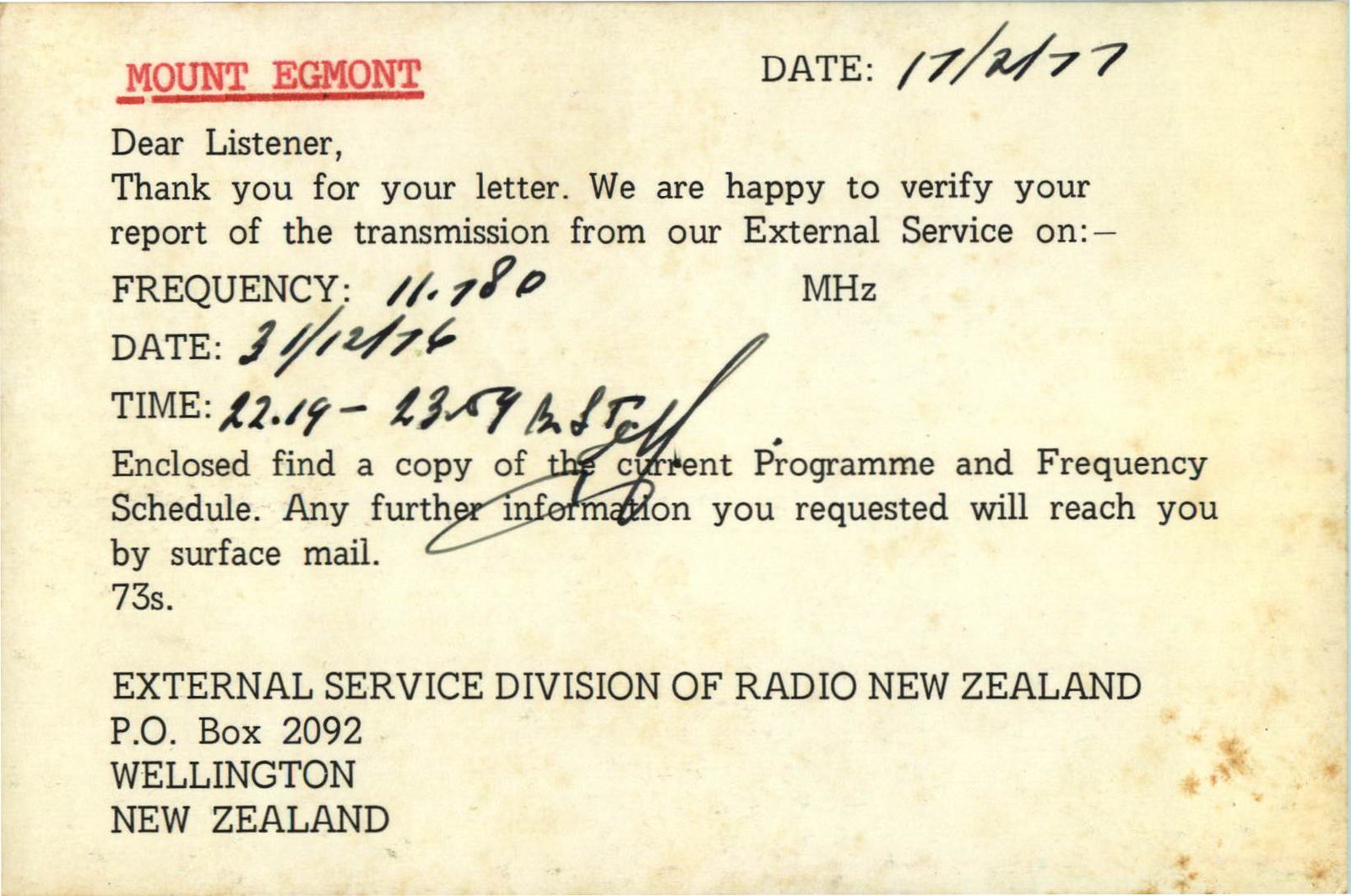The image depicts an old, yellowed postcard with visible age spots and discoloration. At the top, in red, it reads "Mount Egmont," followed by the date "17/2/77" in black capital letters. Below this, typed in a typewriter-style font, is a message: "Dear Listener, Thank you for your letter. We are happy to verify your report of the transmission from our external service on frequency 11.780 MHz. Date 31/12/76. Time 22:19 - 23:59." There's an illegible signature beneath this text. Further down, it states, "Enclosed, find a copy of the current program and frequency schedule. Any further information you requested will reach you by surface mail. 73s." At the bottom, in large capital letters, it reads, "External Service Division of Radio New Zealand, P.O. Box 2092, Wellington, New Zealand." The card has mold and dinginess, particularly on the right side, adding to its aged appearance.